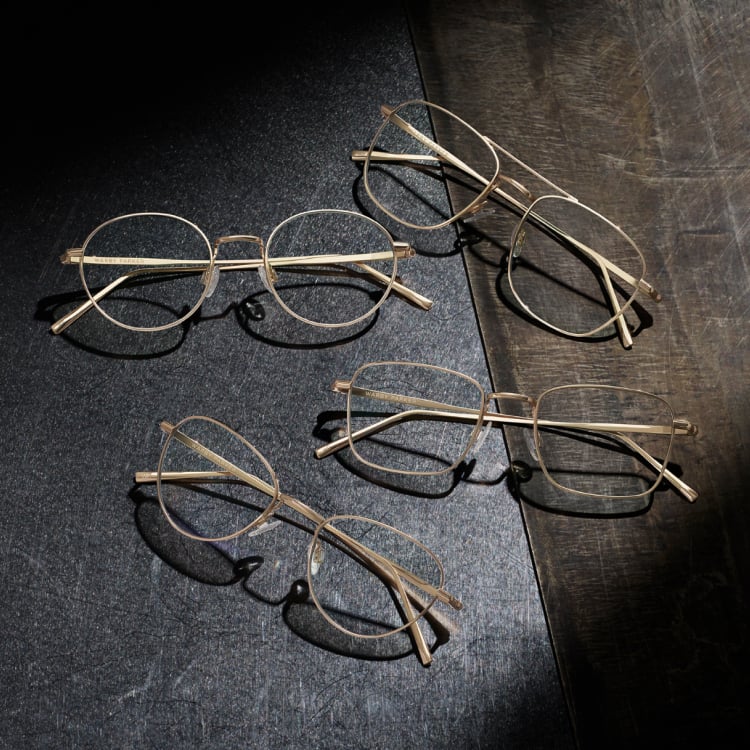The image features four pairs of spectacles, each with frames that appear to be either gold, bronze, or tin-colored. The glasses are neatly arranged on a mixed media surface, which seems to comprise a piece of gray soapstone with white graining on one side and a brownish board with gray undertones on the other. Lit from above, the spectacles cast intriguing shadows on the surface, adding depth to the scene. Two pairs of glasses have circular frames, while the other two have square frames, suggesting a mix of male and female designs. All the glasses are folded and positioned facing upwards, as if neatly placed at the end of a day's use. The background shows some darkness with shadows in the bottom right and top left corners, indicating an interior setting, possibly a house or office.